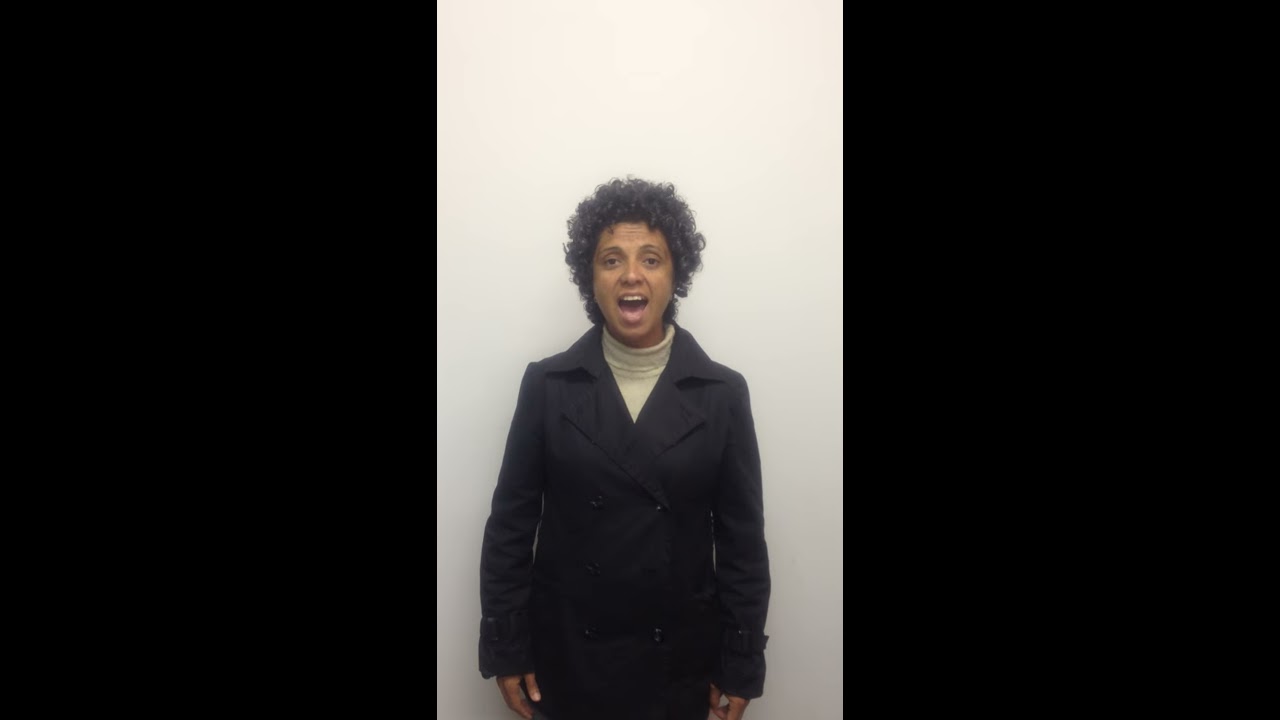The image captures a portrait of a younger woman who appears to be of Indian or Puerto Rican descent, characterized by her light brown skin and curly black hair. She is wearing a cream-colored off-white turtleneck sweater under a black trench coat with large buttons on the chest and a prominent collar. Her arms are resting by her sides, with her hands emerging from the coat sleeves, showing white fingernail polish. The woman has her mouth open, revealing her top teeth in an expression that suggests she might be singing or vocalizing, with her eyes open and face slightly wrinkled, giving it a lively aspect. She is standing in front of a crisp white background, and her figure is centrally framed, creating a striking contrast against the monochromatic backdrop.